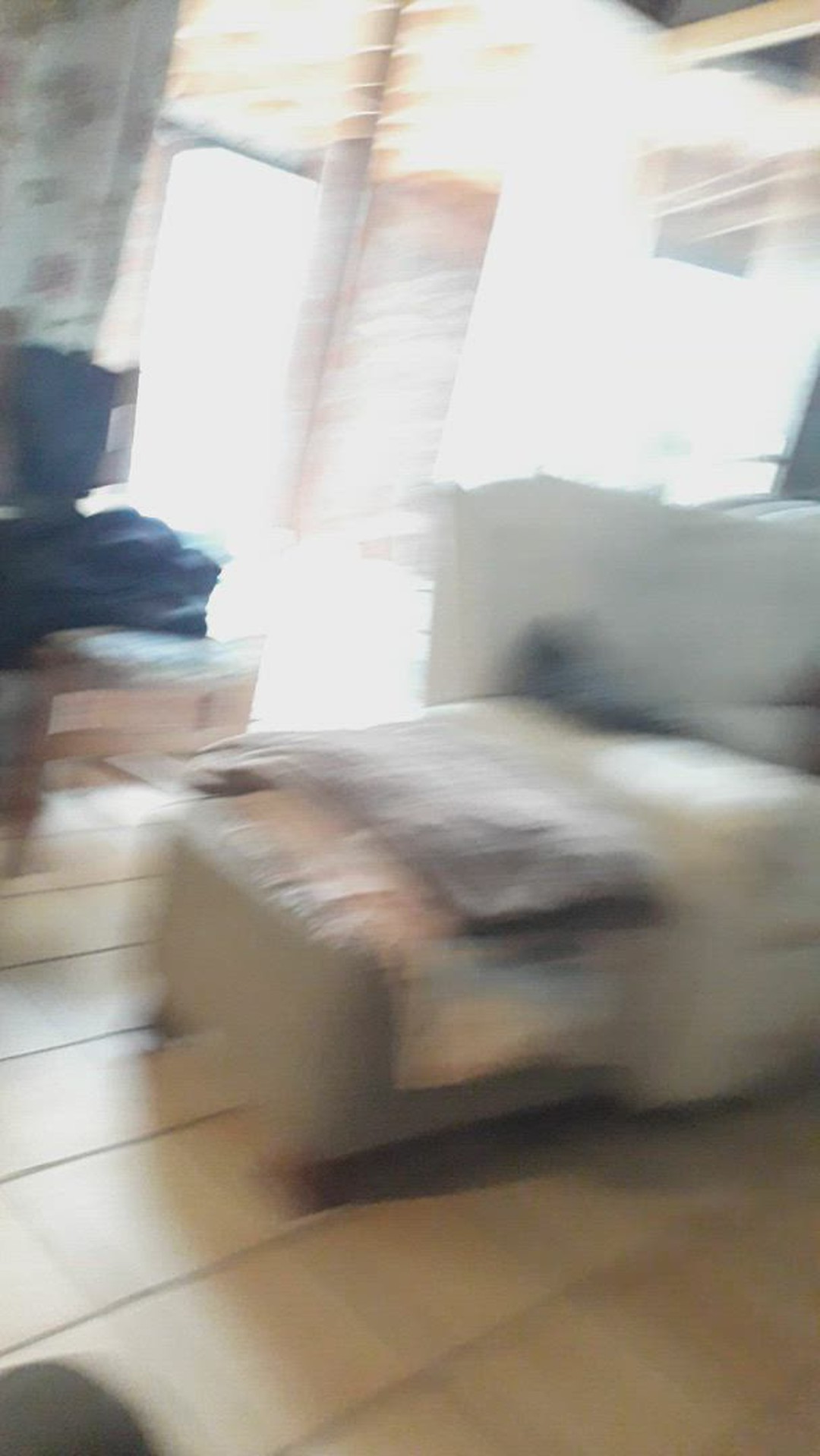This photograph, taken in a blurry, slightly unfocused manner, captures the interior of a cozy room. The ivory tiled floor, with its neatly defined grout lines, forms the foundation of the scene. Prominently placed in the center is a gray upholstered ottoman with short wooden legs, topped with a stack of various fabrics. To the right of the ottoman sits an armless gray upholstered couch, where the bottom and back cushions are partially visible. In the background, against the wall, a computer setup can be seen, its screen clearly positioned near an open door through which warm light streams, adding a soft glow to the ambiance. The composition, though blurred, suggests a comfortable and lived-in space.